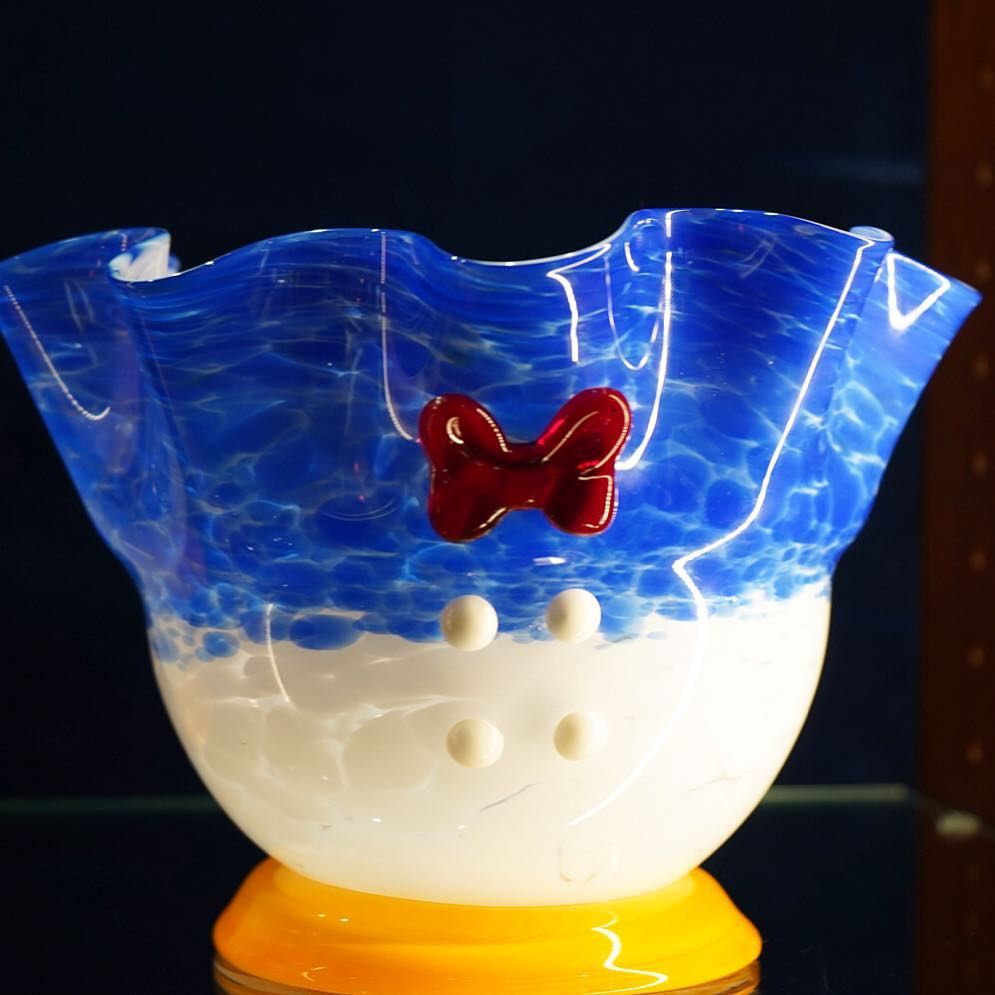This is an indoor, full-color photograph featuring an ornately designed decorative glass bowl under artificial lighting, set against a stark black background. The square image reveals a highly stylized bowl, prominently resting on a vibrant yellow, shiny, saucer-like base. The bowl itself exhibits an artistic blend of colors and textures: the lower half is crafted from solid white glass with four protruding glass dots, two positioned against the white section and two against the blue above. Transitioning upwards, the bowl displays a striking blue hue that is adorned with thin, reflective lines reminiscent of sunlight dancing on water. The bowl's upper lip undulates in a wavy pattern, enhancing its artistic flair. Adding a focal point to the design, a red glass bow tie (or possibly a butterfly) is affixed near the junction of the white and blue sections. The entire piece appears as if it were a meticulously blown glass artwork rather than a utilitarian object, emphasizing its decorative purpose. Nestled in the lower portion of the image is a conspicuous white vertical line, and to the right, hints of wooden elements suggest the photograph was taken in an indoor setting, possibly near a shelf or doorway.